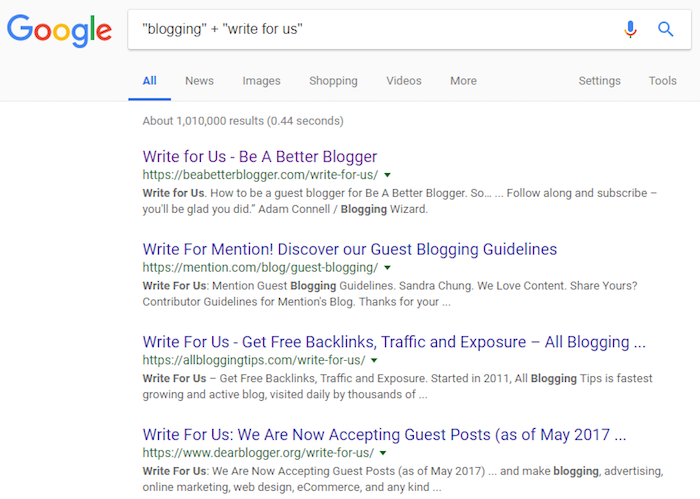The image depicts a Google search results page. At the top left corner, the Google logo is prominently displayed. To the right of the logo is a long white rectangular search bar, inside which is the search query "blogging" + "write for us". Adjacent to the search bar on the right, there are two icons: a microphone icon and a magnifying glass icon. 

Below the search bar, there are six categories starting from the left: "All," which is highlighted in blue, followed by "News," "Images," "Shopping," "Videos," "More," with "Settings" and "Tools" located on the far right, all in gray text. Underneath these categories, the page indicates that there are about 1,010,000 results for the search query.

The top search result is titled "Write for Us - Be a Better Blogger" with the website link "beabetterblogger.com" immediately below it. The accompanying sentence provides additional details about the website. The second result is titled "Write for Mention! Discover Our Guest Blogging Guidelines," with the website link "mention.com" in green. The third result is "Write for Us - Get Free Backlinks, Traffic, and Exposure," directing to "allbloggingtips.com." The final result on the page is "Write for Us - We Are Now Accepting Guest Posts," and the website link is "dearblogger.org."